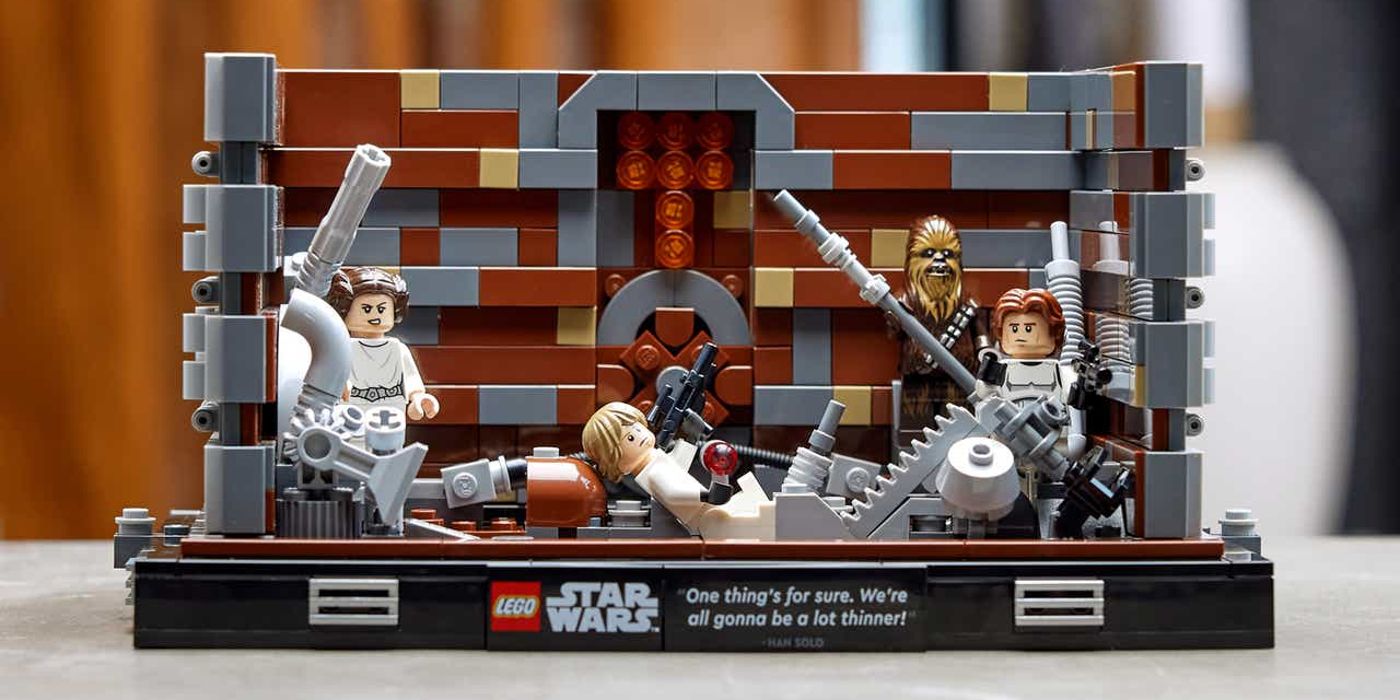The image showcases a meticulously assembled Star Wars Lego set depicting a scene from the first movie where the characters have fallen into a junk area. The diorama features Princess Leia standing in the left corner, Chewbacca and Han Solo in the right, and Luke Skywalker lying on his back in the middle, leaning against some debris. Han Solo is notably wearing a stormtrooper outfit without the helmet, while Chewbacca faces the viewer, clutching a large pole. The walls of the junk area are constructed from brown and gray Lego blocks, creating a confined, cluttered scene true to the film. The bottom of the image highlights the Lego logo in a red square with white font, accompanied by "Star Wars" in white and the quote "One thing's for sure. We're all going to be a lot thinner." This detailed set captures a pivotal moment with all the iconic characters and their weapons, reflecting a true-to-story Star Wars experience.